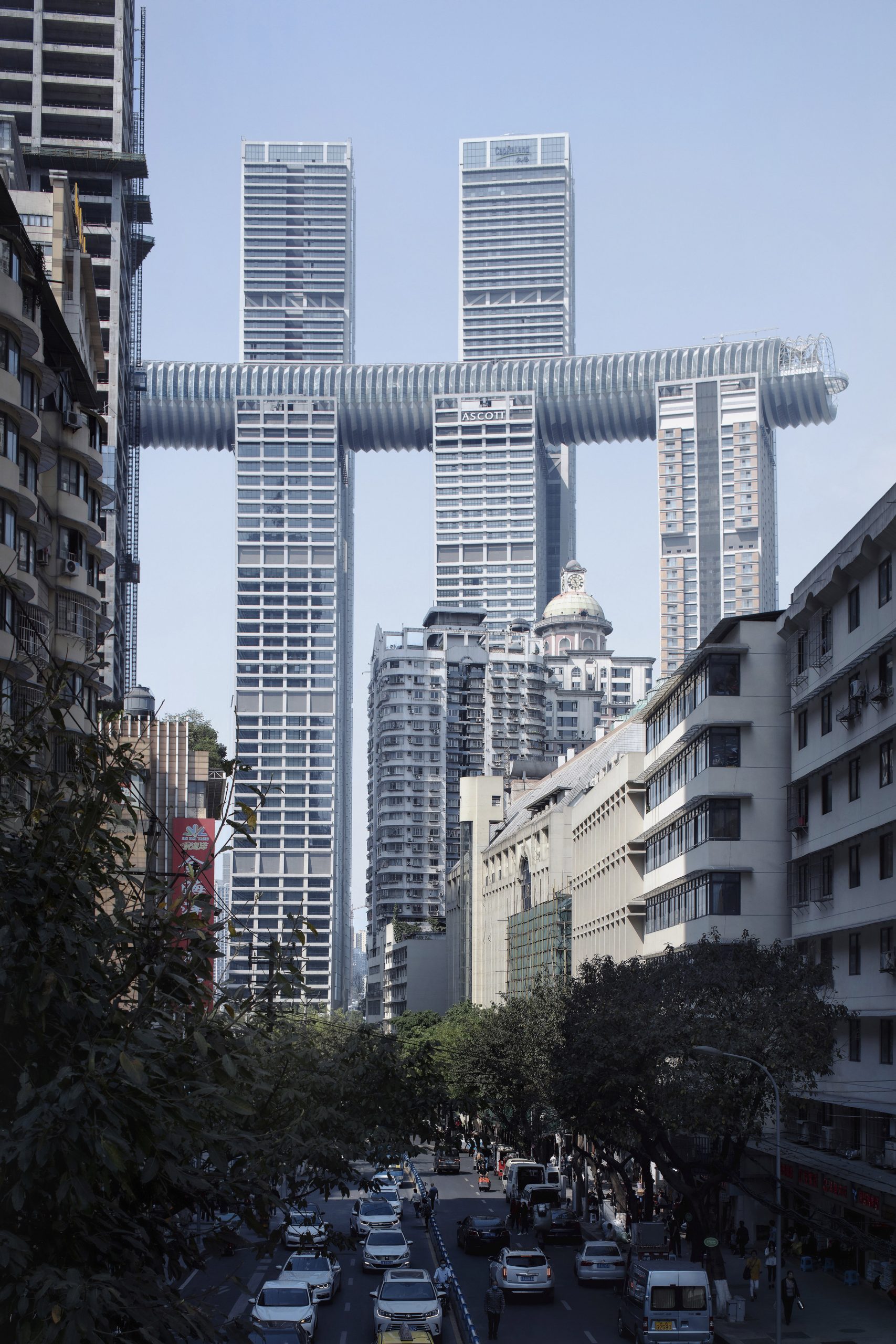The image captures a bustling outdoor city scene, characterized by numerous tall office buildings and skyscrapers against a light blue sky. Dominating the background are two exceptionally tall, straight, skinny buildings, with a distinctive round, tube-like sky bridge connecting them. In front of these towering structures are three slightly shorter buildings, their tops connected by a coiled, straw-like gray piece with the word "Ascot" prominently displayed in the middle. The foreground reveals a busy four-lane street filled with numerous white cars and lined with trees. Sidewalks are populated with people, and the traffic is heavier on the left side. Additionally, smaller high-rise residential buildings flank the scene, each about six to eight stories high. A green, leafy branch extends across the center of the photograph, adding a touch of nature to the urban setting.